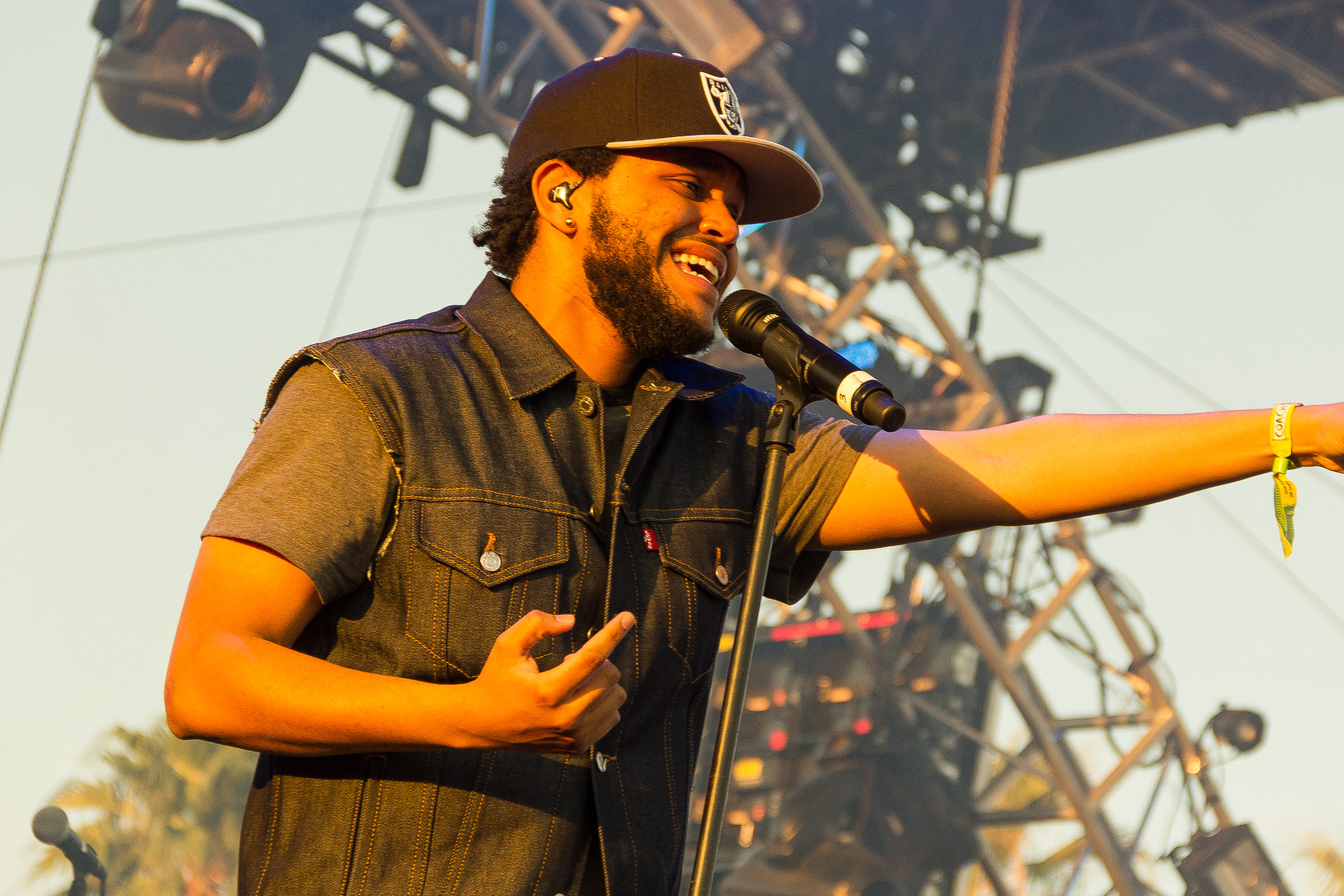In the image, we see a performer on stage who bears a resemblance to either The Weeknd early in his career or the singer from Gym Class Heroes. He is a man of likely black or mixed heritage, wearing a black cap emblazoned with the Raiders logo. The performer listens to music or cues through earbuds and is dressed in a distinctive denim vest with frayed sleeves that appears to be from Levi's, as indicated by the visible red tag. Underneath the vest, he sports a gray t-shirt. His left wrist is adorned with a yellow Coachella festival wristband, typically issued to attendees. Despite his arm being slightly cut off in the photograph, he seems to be engaged with the audience through a gesture. The background is filled with scaffolding and stage equipment, setting the scene of a concert or festival.